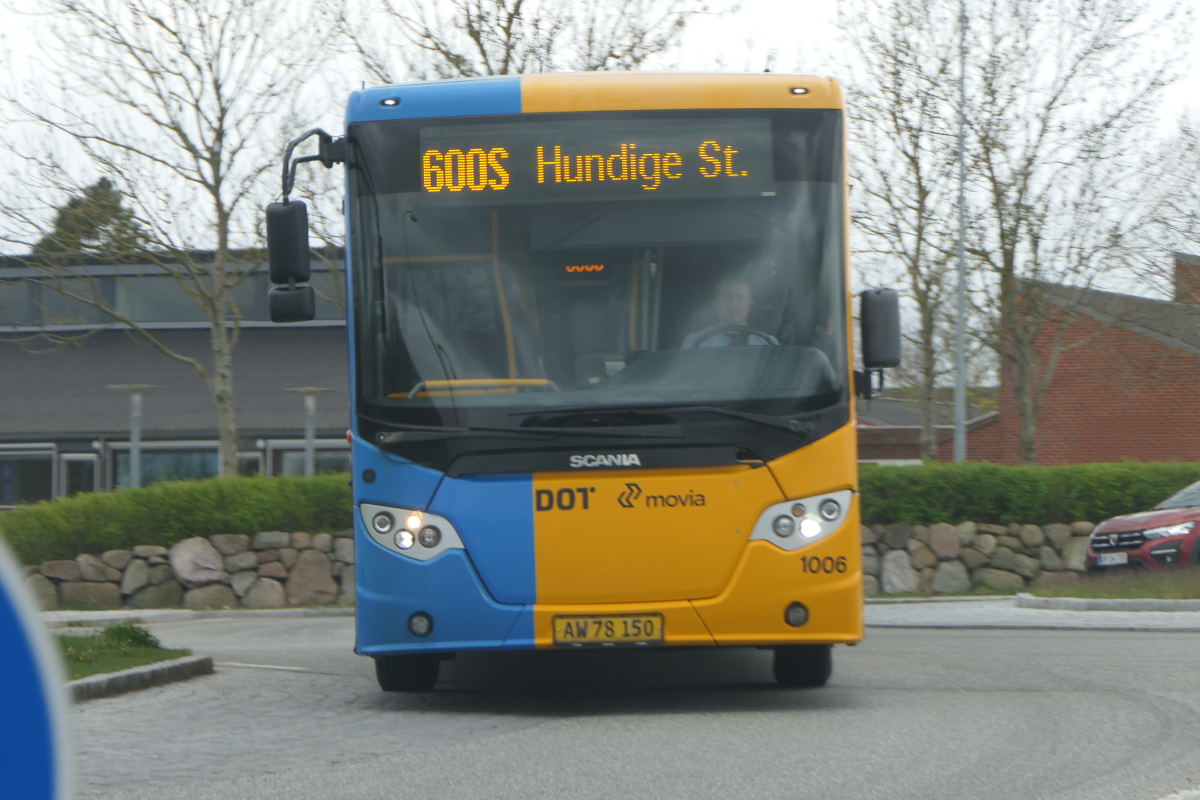This detailed photograph captures a head-on view of a bi-colored public transit bus, prominently featuring its blue left side and mustard yellow right. The bus displays "600S Hundige Street" in yellow letters across the top electronic marquee sign. The windshield, encased in a black border, shows "Scania" in silver lettering, "DOT" in black, and "Movia" beneath it. The bus, marked with the number 1006 below the right headlight frame, has a yellow license plate reading "AW78150". The middle-aged, white male driver, donned in a blue shirt, navigates around a roundabout, with a red Impala trailing him. This scene is set against the backdrop of bare trees—likely poplars—hinting at autumn, along with two prominent buildings: a red brick structure with a gray roof and a dusty old gray building to the left. The area is bordered by stone walls topped with green bushes, and the overcast, light-gray sky underscores the season.